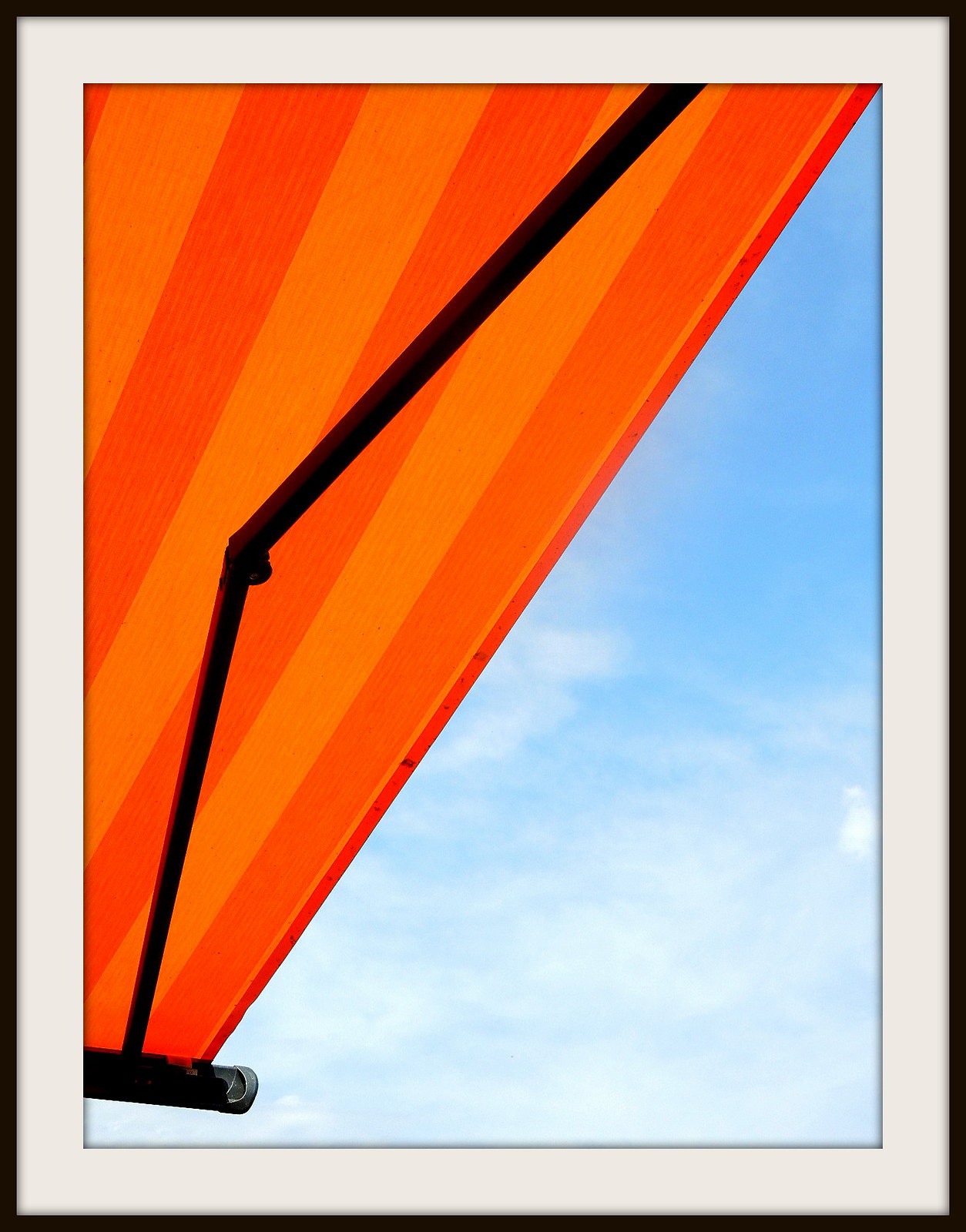In this image, a roll-out awning with vibrant stripes of dark and light orange extends elegantly into the frame. A single fold-out, crank-operated support arm, nearly fully extended, holds the awning in place. This style of awning and support is typically found attached to trailers in campgrounds or on building edges, suggesting its portable and retractable nature. Beyond the awning, the sky is a stunning canvas of deep blue adorned with fluffy, hazy white clouds, adding a serene, picturesque backdrop to the scene.